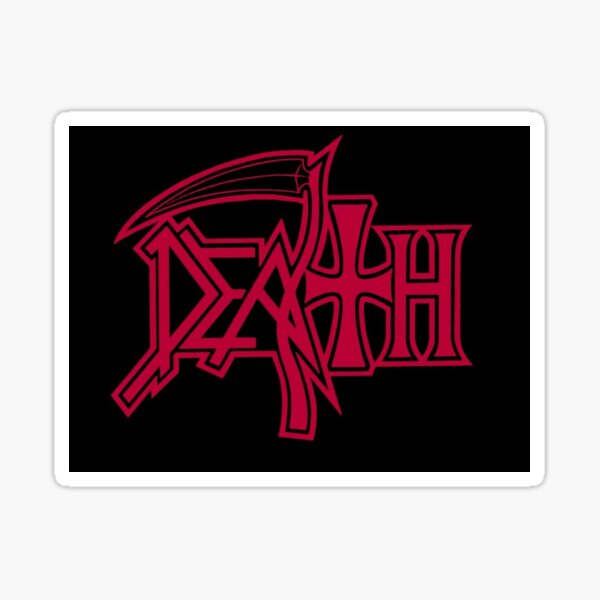The image features the word "Death" stylized in a striking, edgy font reminiscent of 1980s metal rock band logos. The word is prominently displayed in a vibrant hot pink color, outlined in black, against a solid black background. Notably, the letter "T" is designed to resemble a Templar cross, emphasizing the grim theme. Between the "A" and "T," there is a sickle, symbolizing a grim reaper's blade. This sickle has a black handle outlined in black, with a pink spine running through the blade. Surrounding the image is a white-colored border, separated from a gray line that frames the entire composition, giving it a framed appearance. This design's punk rockish elements and detailed accents create an intense, visually striking logo.